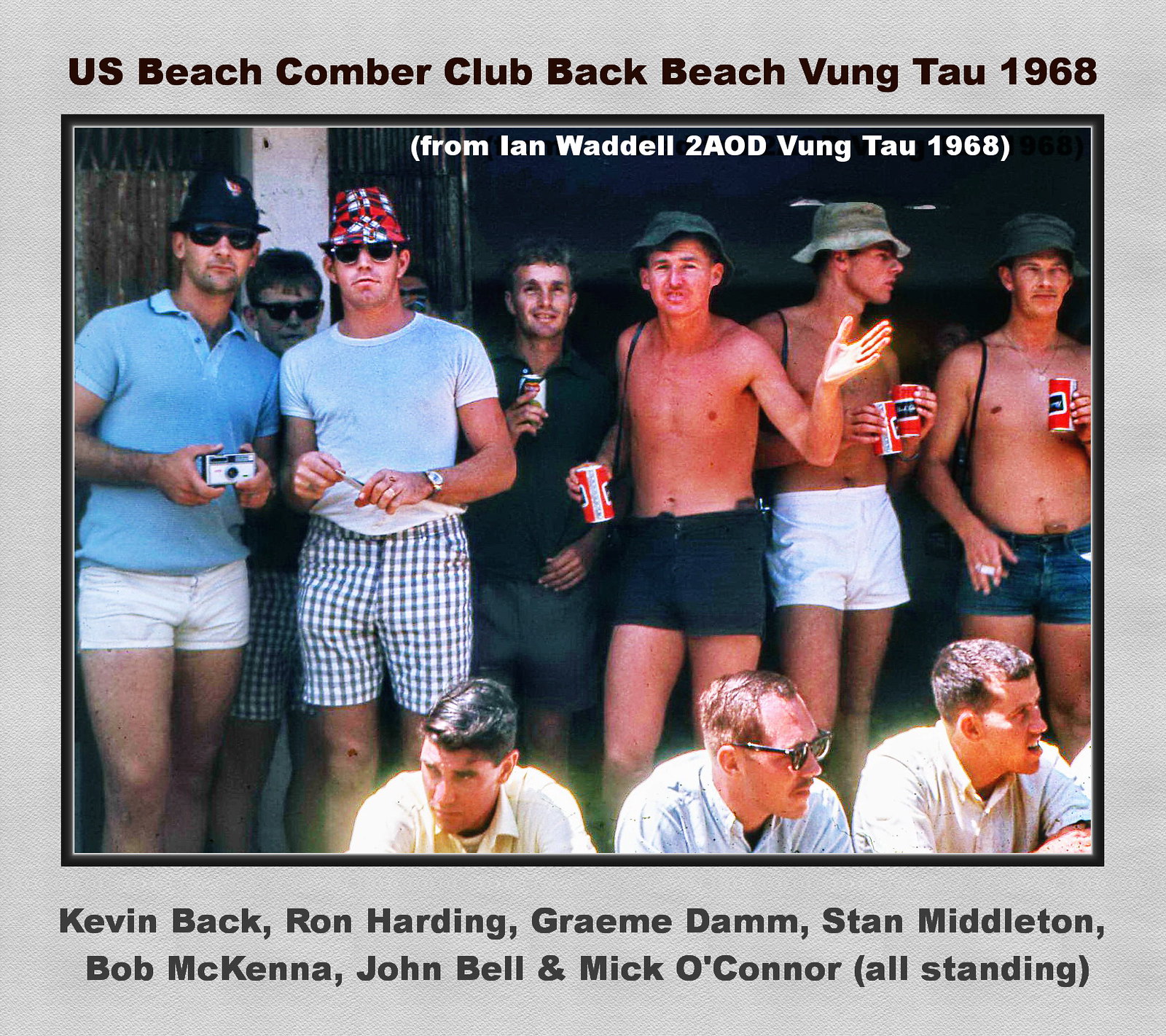The photograph depicts a group of men, mostly in their 20s, partaking in a social gathering at the U.S. Beachcomber Club, Back Beach, Vung Tau, in 1968. At the top of the image, the caption reads, "U.S. Beachcomber Club, Back Beach, Vung Tau, 1968." Also inscribed at the top is a note, "From Ian Waddell, 2AOD, Vung Tau, 1968." Below the group, the names of the individuals are listed: Kevin Buck, Ron Harding, Graham Dam, Stan Middleton, Bob McKenna, John Bell, and Mick O'Connor, all standing.

The leftmost man wears a blue t-shirt and dark glasses, holding a small camera across his chest. Most of the men wear bathing suits, with three of them shirtless, sporting floppy hats in various shades including blue, gray, and off-white. Several men are holding cans of beer, identifiable by their vertical white and red stripes. One man's cap is decorated with red flowers, while others wear green and black caps.

In the foreground, three men sit, dressed in dress shirts, with one wearing sunglasses. The scene captures a moment of camaraderie and leisure among the men, distinguished by their casual attire, shared beverages, and relaxed demeanor.